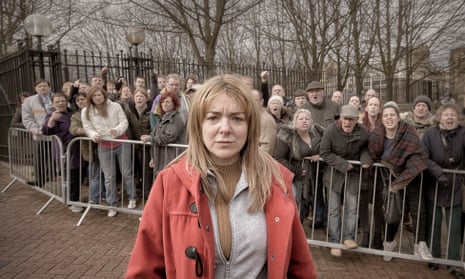This image captures an intense protest scene during the fall or midwinter season. The setting is outdoors, with barren trees and light posts in the background indicating a cold, leafless time of year. Central to the image is a distressed woman with long, blondish hair, who stands on a brick path in front of a large group of approximately 30 people crowded behind a waist-high, movable metal fence. 

The woman, positioned at the forefront and center of the photo, is layered against the cold in a reddish jacket over a white zip-up jacket, both atop a golden brown turtleneck sweater. Her facial expression is tense, with a furrowed forehead, while the crowd behind her appears agitated, yelling or shouting with visible frustration. The overall mood of the scene is dark and intense, with no one showing signs of happiness.